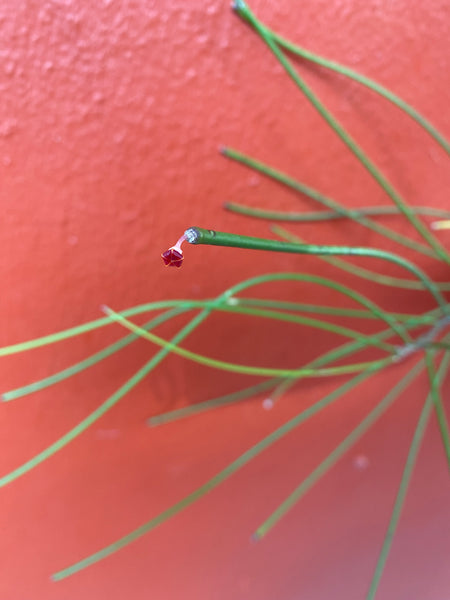The image showcases an extremely close-up shot of what appears to be artificial artwork, dominated by a textured pink or salmon-colored backdrop, possibly resembling a painted stone wall. Emerging from this vividly colored background are several long, green, wire-like stems, resembling plant tendrils or green onions. One prominent stem in the foreground, which is notably distinct, appears to be cut, revealing its internal structure and giving the impression of an unripened bud at its tip. The lifelike yet synthetic texture of these green projections emphasizes their artificial nature, evoking a sense of manufactured vegetation against the pinkish canvas. The overall composition focuses on the intriguing contrast and detail of the green projections against the textured, colorful backdrop.